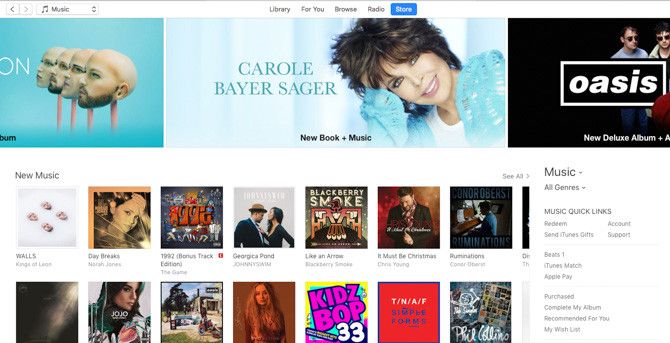The image displays a user interface resembling the Apple Music or iTunes application. In the upper left corner, there is a clickable button featuring a music note with the label "Music." The top navigation bar includes tabs for "Library," "For You," "Browse," "Radio," and "Store," with the "Store" tab currently highlighted in blue.

Displayed prominently are images of featured artists. In the center, an image of Carole Bayer-Sager is shown, depicting her with brunette hair, wearing a blue shirt over a white undershirt, and resting her hand on her head. To the right, there is a black-and-white image labeled "Oasis," featuring three men wearing glasses. To the left is an artsy image with a turquoise background displaying four human heads in close-up.

Below the featured artist images, the interface lists various sections such as "New Music," "Music to the Right," and "All Genres." Quick links available at the bottom include "Account Support," "iTunes Match," "Apple Pay," "Purchase," and "Complete My Album." Overall, the display seems to offer an overview of the latest music releases and the general layout of the application, reinforcing the likelihood that this is an Apple Music or iTunes window.